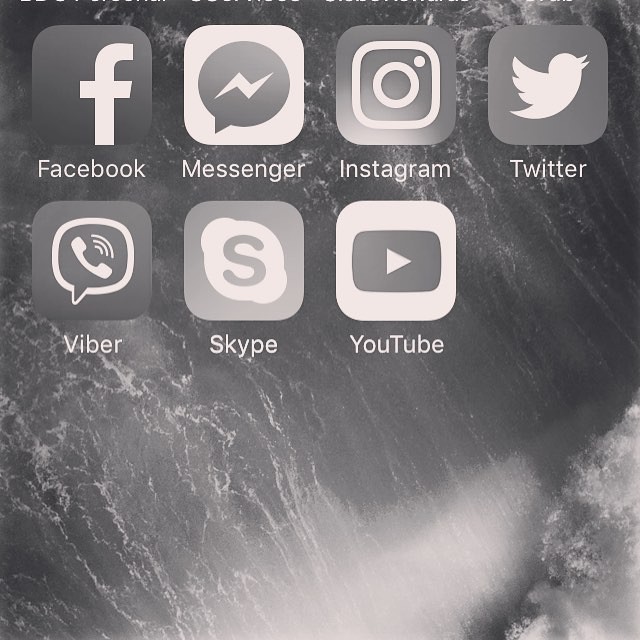This black and white image captures a portion of a smartphone screen, specifically the upper half, showcasing seven commonly used apps arranged in a grid. The image is monochromatic, adding a timeless aesthetic to the screen's display.

1. **Top Row (Left to Right)**:
   - **Facebook**: The icon features a bold 'F' with the label "Facebook" beneath it.
   - **Messenger**: Displayed as a speech bubble with a zigzag line, and labeled "Messenger."
   - **Instagram**: Represented by a square icon with a circular camera design and a dot, labeled "Instagram."
   - **Twitter**: The iconic silhouette of a bird facing to the right, labeled "Twitter."

2. **Bottom Row (Left to Right)**:
   - **Viber**: A speech bubble icon featuring an old-school phone receiver with three arched lines indicating a ring. The label reads "Viber."
   - **Skype**: Identified by a round icon with two bulges on the top left and bottom right, containing an 'S' in the center, labeled "Skype."
   - **YouTube**: The classic rectangle with a play button (triangle) facing to the right, labeled "YouTube."

The background image of the phone screen depicts a mesmerizing waterfall. The close-up shot emphasizes the flowing water with visible spray at the top right corner, adding a dynamic element to the otherwise static arrangement of app icons.